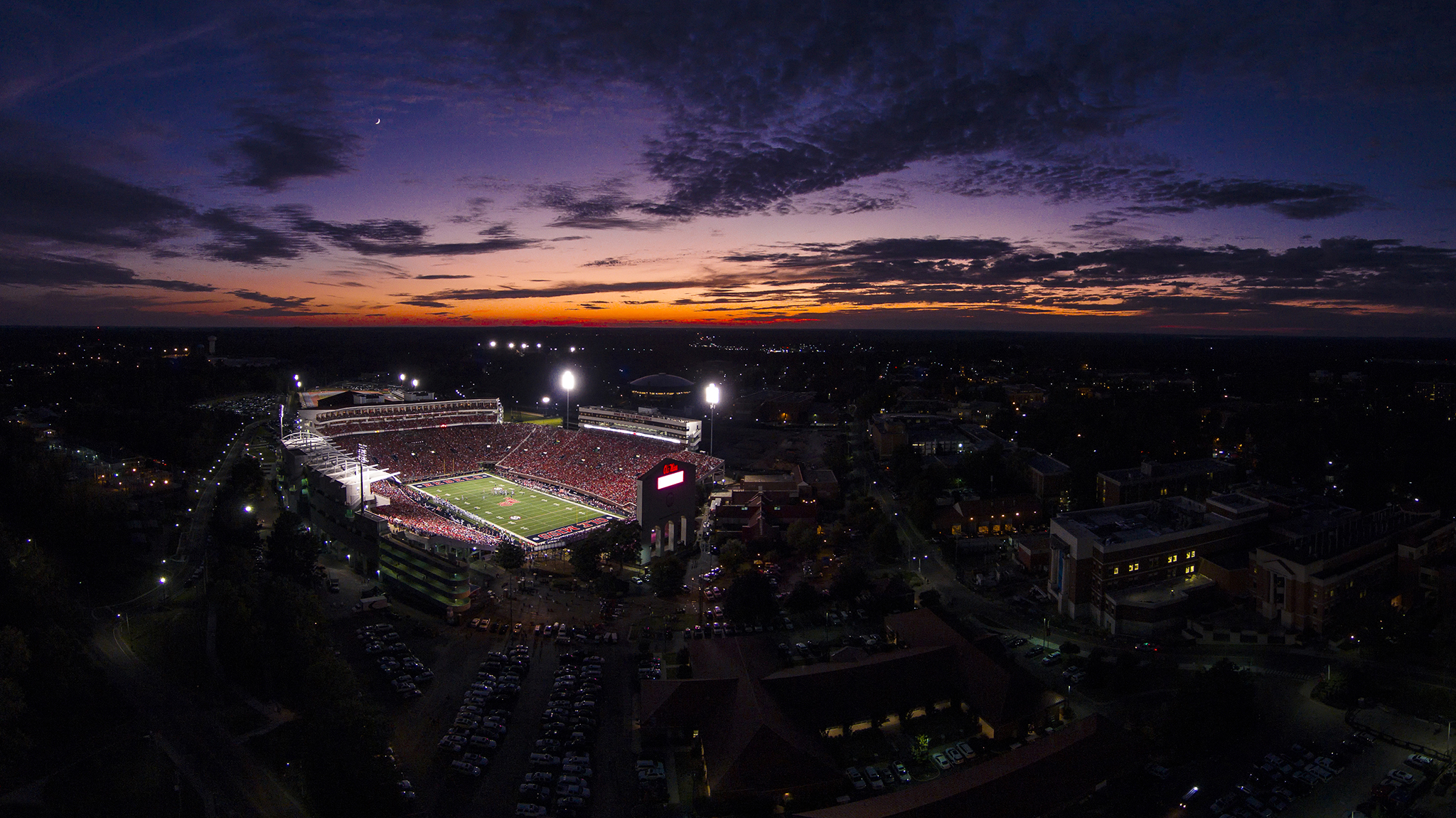From a high vantage point, this aerial shot captures a bustling stadium at dusk, nestled in the midst of a darkened city. The sky transitions into deep purples, blues, and almost black as the sun sets, leaving an orange and yellow haze on the horizon. Dark clouds loom above, enhancing the dramatic twilight. 

In the center of the image, the well-lit stadium stands out prominently. The bright, stadium lights illuminate the green football field below, where a few players can just be seen moving. The towering spectator stands are filled with a multitude of people, appearing as tiny dots against the grand structure. Surrounding the stadium, parking lots are packed with cars.

The city around the stadium is a canvas of silhouettes, with buildings and streets faintly visible due to the lit windows and scattered street lamps. An intersecting network of streets can be seen, with some medium-sized buildings in the foreground, their windows emitting a warm glow. A digital sign on the stadium, glowing with white and red light, adds a final touch to this vibrant scene.